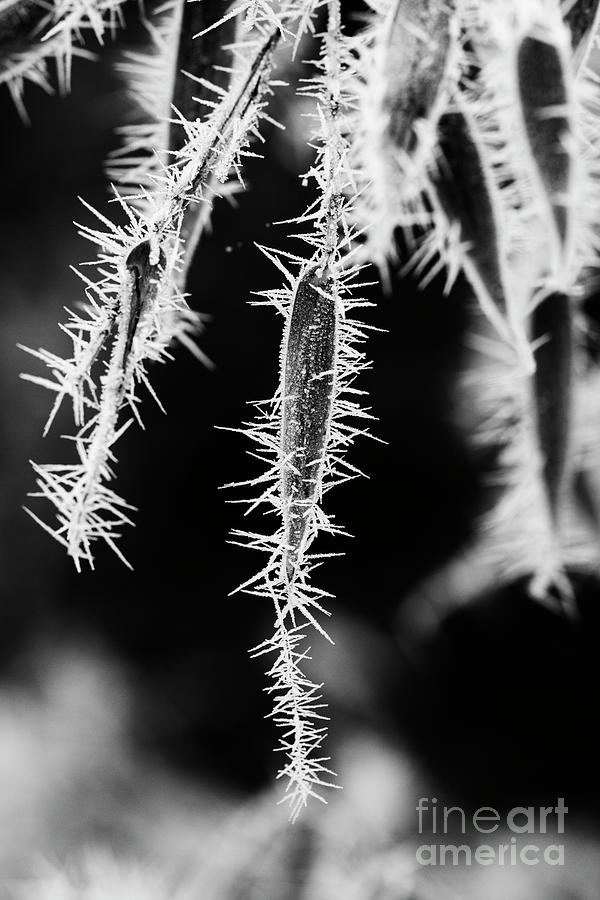This highly detailed black-and-white photograph captures a close-up view of what appears to be elongated, snow-covered leaves or possibly seed pods, adorned with frost spikes. These frosted tendrils cascade downward like streamers from a cactus, intricately spaced and giving a delicate, almost ethereal appearance. The focal point of the image is on these frost-laden, hanging elements, showcasing their sharp, crystalline details, while the background fades into a subtle blur, enhancing the contrast and depth. The lower right corner bears the logo of Fine Arts America, written in a transparent gray font with "fine" in regular lettering, "art" bolded, and "america" in lowercase, grounding the stunning natural scene with a touch of artistic branding.